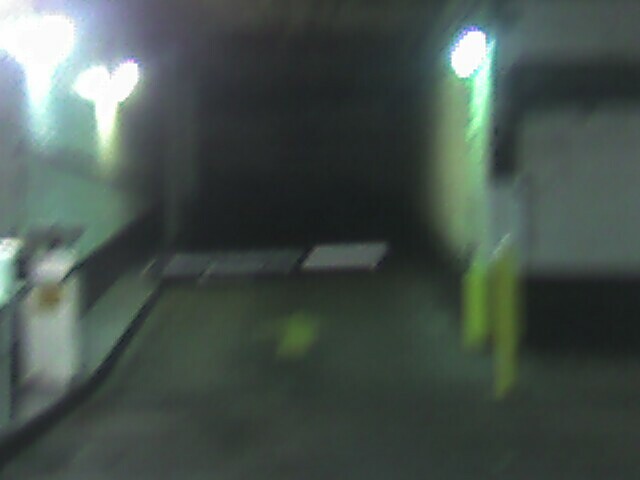A heavily blurred photograph of the interior of a parking garage. The scene is dominated by a cement floor and is punctuated by yellow pylons that line the pathway. A yellow arrow is visible on the ground, suggesting a direction towards either an exit or an entrance. An indistinct object, possibly a barrier arm, stretches across the image, likely controlling the flow of vehicles. To the left, there appears to be a counter, though the lack of clarity makes it difficult to discern specific details. The image is predominantly in shades of black, gray, and white, with bright lights illuminating the space and casting reflections on the walls. The entrance of the garage merges into the background amidst the blur.